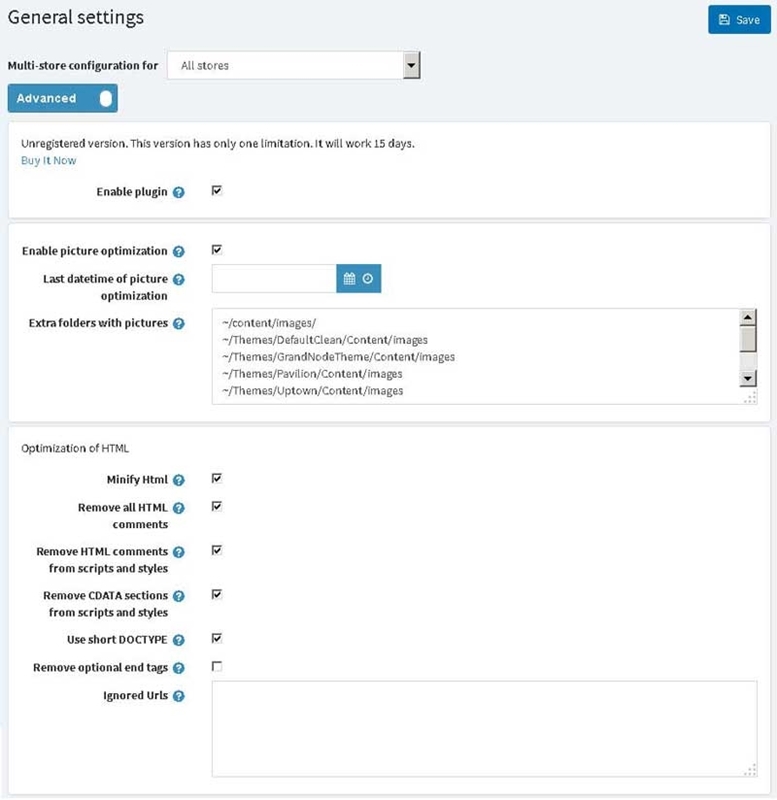This screenshot showcases the General Settings menu of a device, which is configured for a multi-store setup. Beneath the multi-store configuration, various advanced settings are listed. Key options displayed include 'Picture Optimization', allowing for refined image display, and 'Date-Time Notification on Pictures,' which likely adds timestamps to photos. Additional settings include the option to 'Remove HTML Comments' and manage 'Extra Folders and Pictures'. Notably, the device is currently using an unregistered version limited to a 15-day trial period. The user has enabled the 'Plug-In' option, as indicated by the checked box, and has also activated 'Picture Optimization'. Furthermore, they have organized extra folders containing images and optimized the HTML settings, enhancing the device's overall functionality.